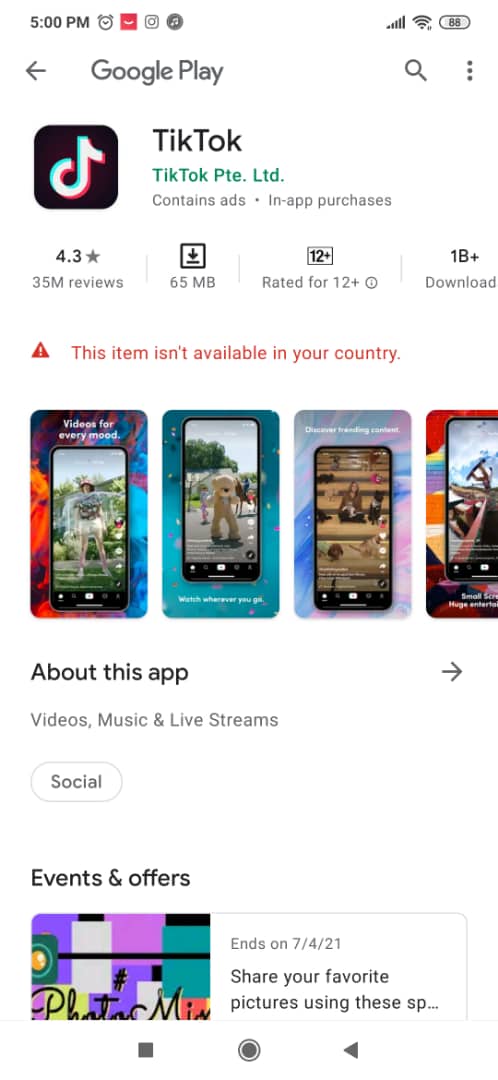The image displays a screen capture taken from a mobile device. The background of the screen is white. In the top left corner, the time is shown as 5 PM. To the right of the time, several other icons are visible. Below the time, large black text reads "Google Play." Directly below "Google Play" on the left side, there is the TikTok icon, which features the TikTok logo in white and black on a black square with rounded corners. To the right of the icon, the word "TikTok" is written in black text. Below that, "TikTok PTE Limited" is written in green. The middle section of the image showcases several images shaped like the front views of mobile phones or devices. These images are displayed in a row from left to right, and vary in color: starting with red and blue, followed by green, then a mix of lilac and blue, and finally red, orange, and yellow.